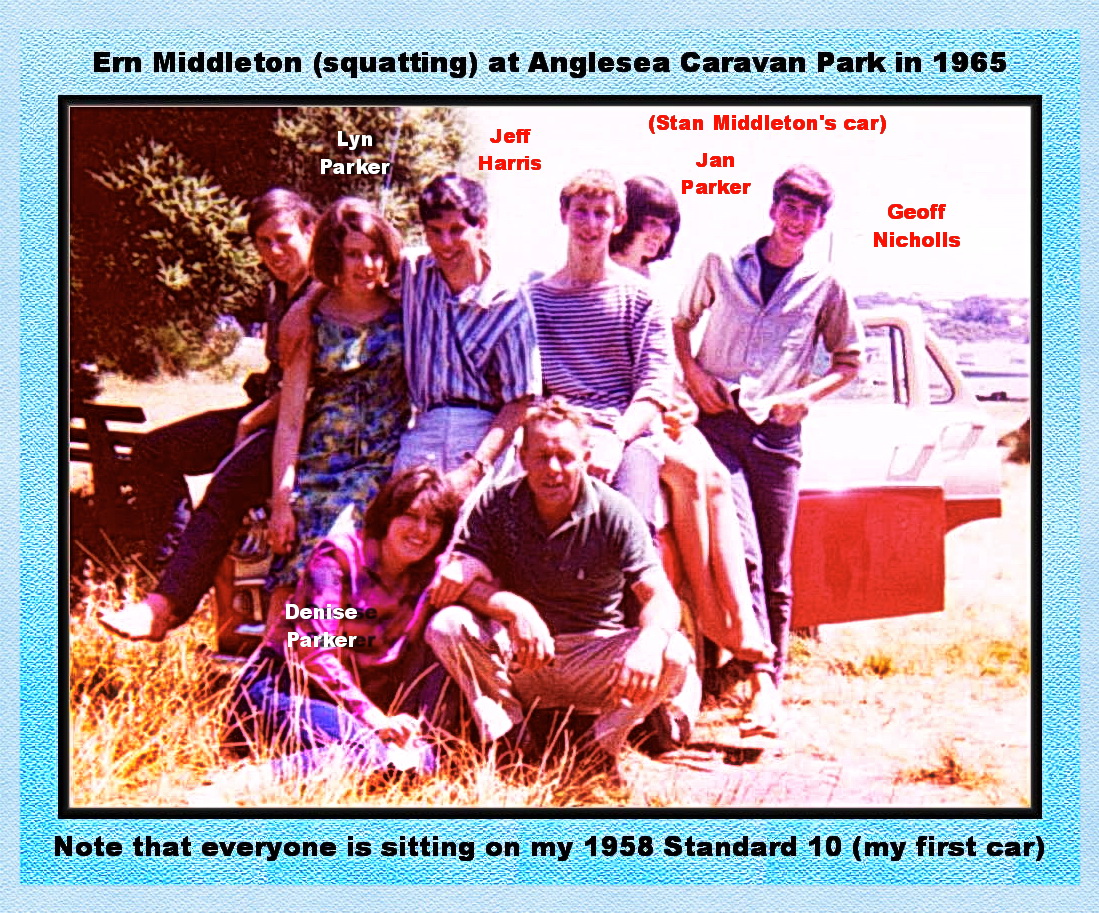In this vibrant photo taken at Jelsea Caravan Park in 1965, a group of eight people are captured enjoying a sunny day outdoors. They are gathered around a red 1958 Standard 10, which is noted at the bottom of the photo as "my first car." Six people are either sitting or leaning against the car, which is set in a weeded area with a tree visible in the upper left. A woman sits on the grass at the front of the group, her arms latched onto a kneeling man who is holding a cigarette and wears a short-sleeved shirt. Another woman in a blue, white, and yellow dress sits on the car. The names of the people are labeled in red and white text: from left to right, Lynn Parker, Jeff Harris, Jan Parker, Jeff Nichols, with Denise Parker at the bottom left. A bench with wood slats is on the left side, and a camper van is visible towards the back right. The sky appears blank, adding a timeless feel to the image. Noteworthy text above the photo reads, "Ern Middleton squatting at Jelsea Caravan Park in 1965," and at the top right, "Stan Middleton's car" is noted in red text.